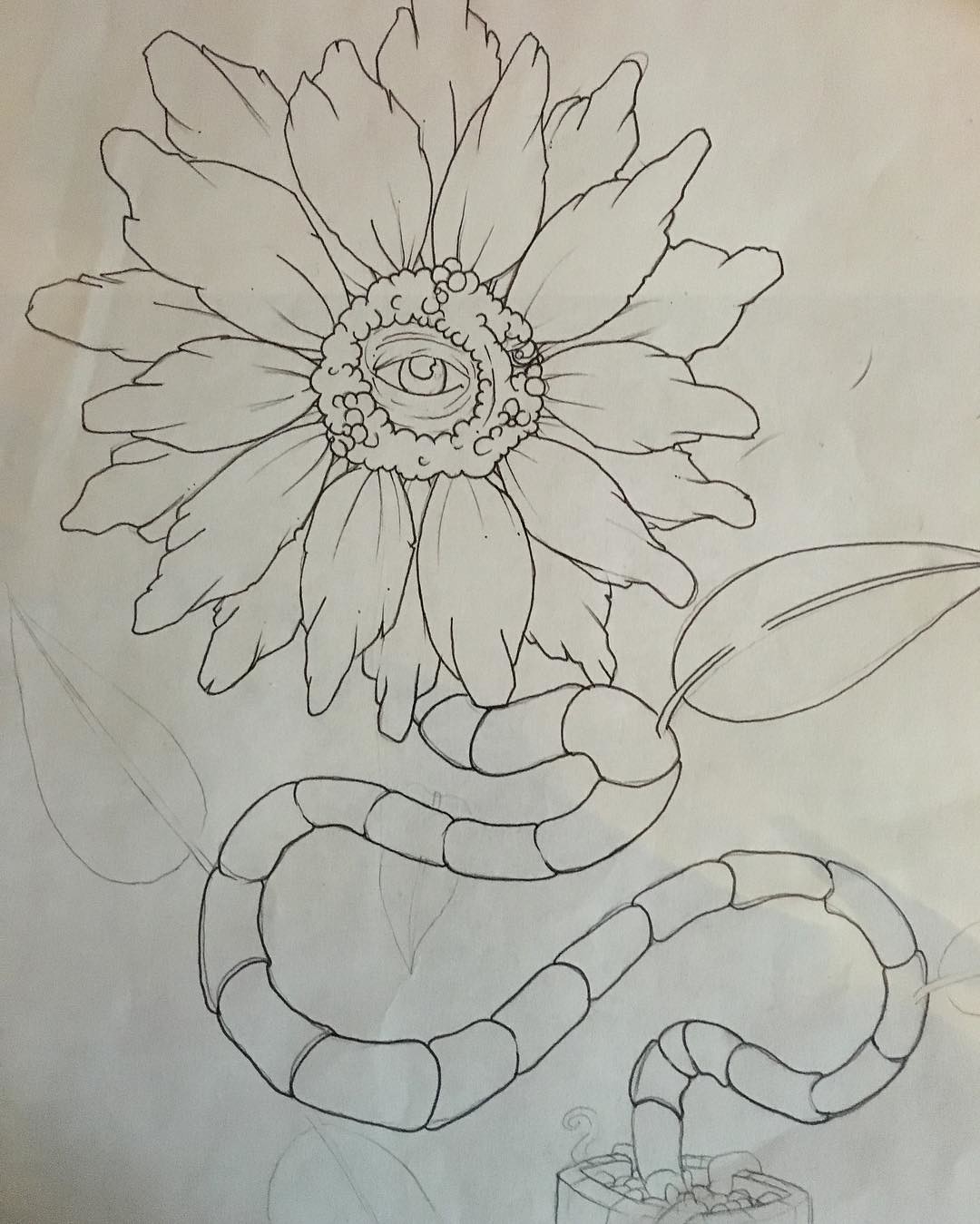This is a photograph of a detailed black-and-white drawing on plain white paper, showing visible creases suggesting it has been folded. The artwork is partially completed and initially drawn in pencil before being inked over. It depicts a fantastical, snake-like plant emerging from a small pot at the bottom, which contains rocks. The segmented, vine-like stem winds upward in a sinuous, swirling manner reminiscent of a snake or worm. A single, fully-formed leaf extends from one side of the stem, while hints of additional leaves remain sketched. The plant culminates in a large, fanned-out flower that resembles a sunflower. However, the center of the flower deviates from the norm, featuring a human eye surrounded by skin-like details within the pollen area, creating an eerie, alien-like appearance.